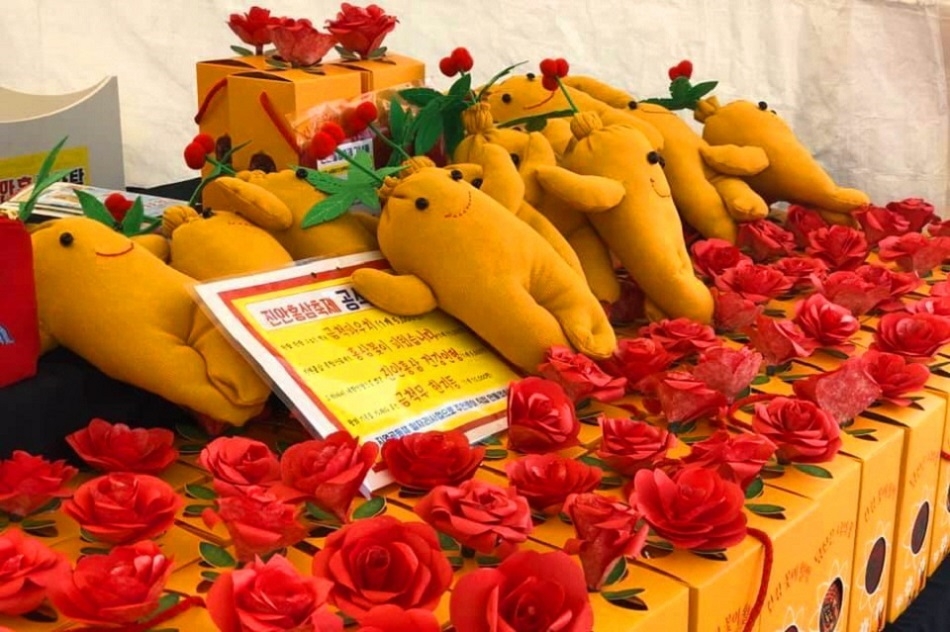The color photograph captures an arrangement of yellow boxes, each topped with red roses and adorned with unique stuffed creatures. These stuffed figures feature minimalistic designs with two eyes, a smiley mouth, two arms, and two legs. Resembling plump yellow carrots with green leaves sprouting from their heads, these adorable characters are arranged in a lively display. In the background, additional yellow boxes with roses extend the scene, and a large sign written in Chinese is prominently positioned at the center. The image also includes a white curtain as a backdrop, enhancing the overall presentation of this quirky and colorful assortment.